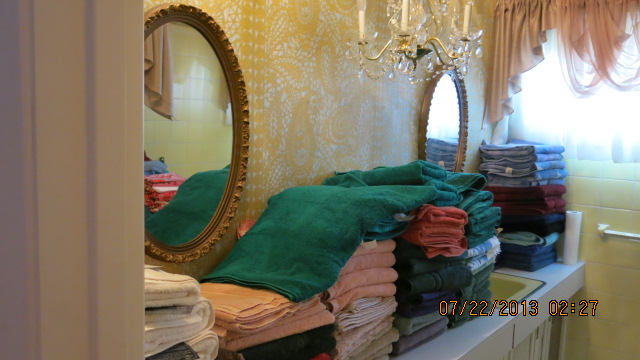This color photograph, dated 07-22-2013 at 02:27, captures an ornate and somewhat dated bathroom interior. The bathroom features a pair of round, gold-framed mirrors above the off-white counters of the vanity, which is flanked by elegantly ruffled pink curtains and further enhanced by the streaming natural light from a window with blinds on the right side. The backdrop is a predominantly yellow paisley-patterned wallpaper with white accents, adding to the vintage ambiance. Central to this luxurious setting is a grand gold and crystal chandelier hanging above the sinks.

The countertop is nearly entirely covered with neatly folded towels, suggesting preparations for a move. These towels come in a variety of mostly dark colors, including greens, maroons, blues, purples, browns, and burgundies, with a few lighter shades like whites, peaches, and grays. This abundance of towels leaves just a hint of the white counter visible beneath them. Overall, the scene reflects both elegance and practical preparation, capturing a moment in the home's history.